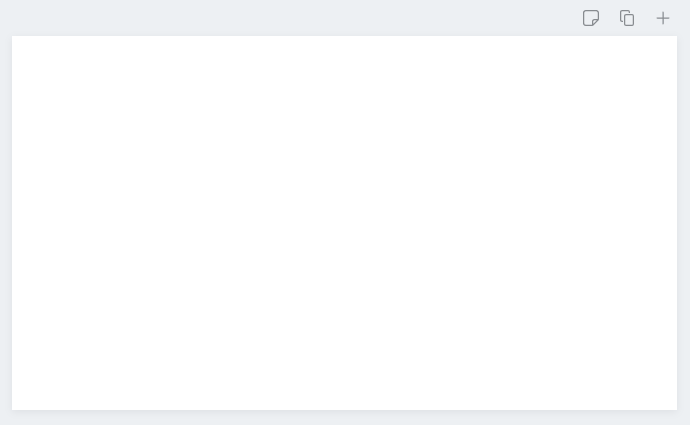**Caption:**

The image features a minimalistic design with a grey-outlined border framing the composition. Located in the upper right-hand corner, a piece of paper, depicted in a darker grey shade, is folded over at the bottom right corner. This paper partially overlays two other pieces, creating a layered effect. Just below and slightly to the left of the folded paper, a prominent plus symbol is displayed. The center of the image remains blank, showcasing a plain white screen devoid of any additional elements.